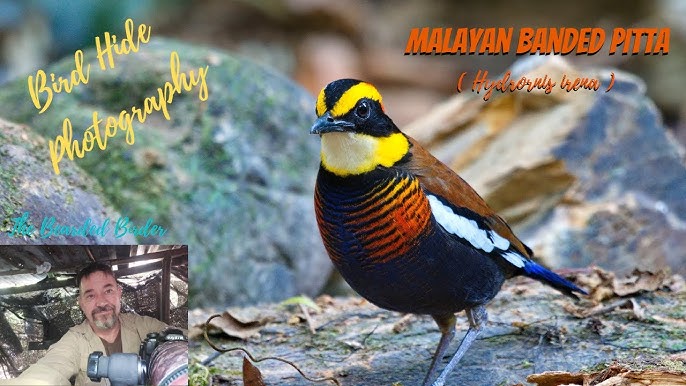This image features an exquisitely detailed Malayan Banded Pitta standing on gray rocks amidst some debris, such as leaves. The bird's vibrant plumage is striking, with a red, black, and blue head adorned with shades of yellow between the top of its head and its black eyes. Cream and yellow hues accentuate the area under its black beak and along its neck. Its body displays rich navy blue tones on the trunk, complemented by reddish, gold, and orange stripes across its chest. The wings are a mix of tannish-red, white, and bright blue, while its tail feathers are predominantly blue. The bird stands on gray feet. 

In the lower left-hand corner of the photo, the photographer is visible, smiling and posing with his camera, seemingly taking a selfie. "Bird Hide Photography" is inscribed in an angled yellow cursive font in the top left-hand corner, while "MALAYAN BANDED PITTA" is prominently displayed in an orange, all-caps font in the top right-hand corner. Beneath this title, another word is italicized, and in parentheses, the scientific name "Hydrornis guajana" is provided, lending a technical touch to the image's description.